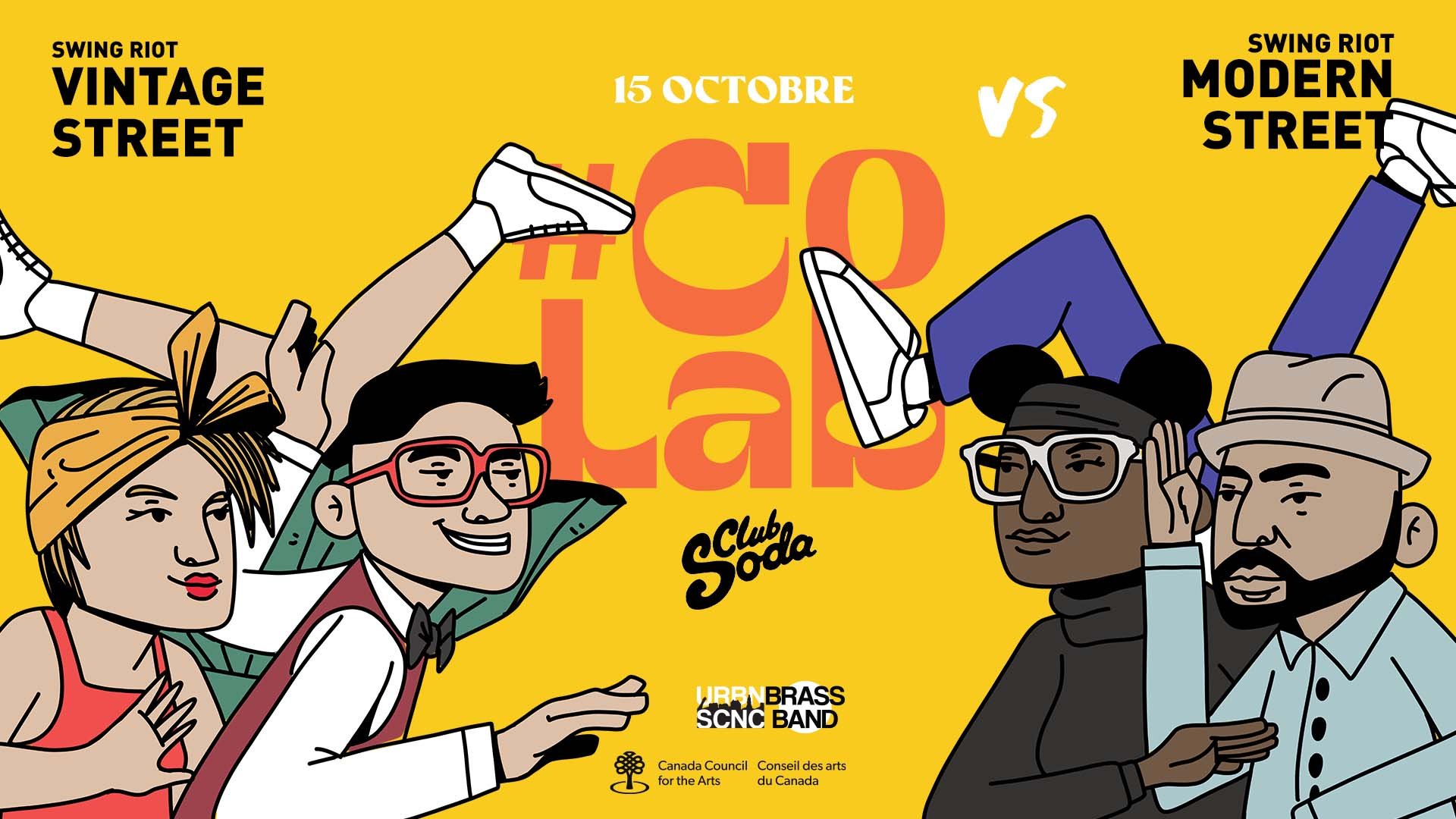The poster, set against a vibrant yellow background, advertises a swing dancing event. At the top left in bold black text, it reads "Swing Riot Vintage Street," while the top right announces "Swing Riot Modern Street." The central portion displays "15th October" in white letters, followed by "VS" and a red vintage hashtag "COLAB." Below, in a smaller cursive black font, it mentions "Club Soda."

The lower half of the image features cartoon figures styled to reflect both vintage and modern themes. On the left, there is a blonde woman with red lipstick, wearing a pink tank top and a yellow bandana, accompanied by a man in a red vest, black bow tie and red glasses. Behind them, a woman in a green dress is mid-air, likely breakdancing. On the right, a black woman sporting space buns and a black turtleneck stands beside a man with lighter skin in a light blue button-up shirt and a hat. A pair of blue pants with white shoes can be seen in the background, illustrating another figure in mid-dance. Between the two groups of characters is a logo for "U-R-B-N Brass S-C-N-C Band" and the "Canadian Council for the Arts," tying together the lively vintage and modern street dance theme.